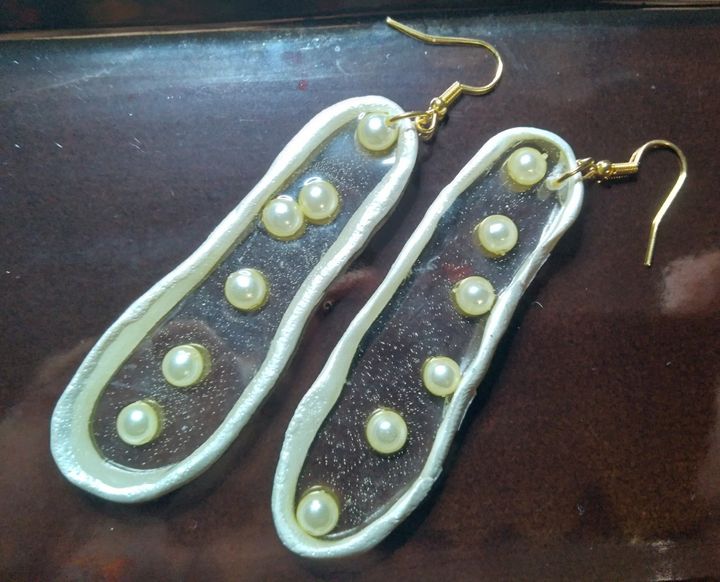The photograph depicts a pair of artistic earrings set on a dark brown wooden table. Each earring features a unique, elongated design shaped somewhat like shoes. They have a flat, translucent base that allows a glimpse of the table beneath, bordered by a thick, white ridge. In the center of the clear insole of each earring are multiple round pearls, arranged differently in each piece. The earring on the left showcases three pearls aligned at the bottom, two placed together above them, and one pearl at the top, making a total of six pearls. Meanwhile, the earring on the right has a sequence of pearls running almost straight downwards, with three positioned in a row and others fanning outward towards the toe, also totaling six pearls. The earrings are equipped with bronze or gold hooks that curve delicately to facilitate wearing. Light from an overhead lamp softly illuminates the table, adding depth to the image and highlighting the intricate details of these elegant earrings.